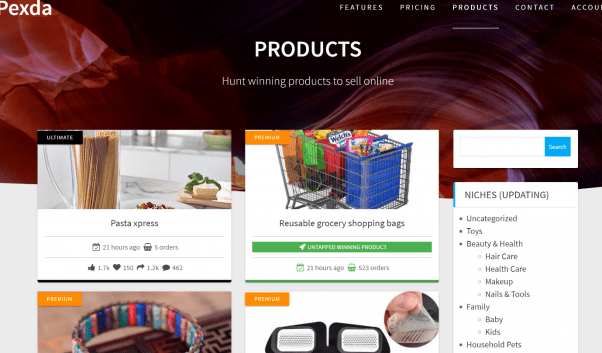The image is an advertisement for a brand named "Hublift," with "Pexter" prominently displayed in white text. The center of the image features the word "Products" in bold, white capitalized text. Below that, a tagline reads, "Hunt winning products to sell online." The background is an abstract 3D rendering of undulating reddish and purplish waves.

At the bottom of the image, various product listings are displayed. The top product is "Pasta Express," highlighted in text accompanied by information stating "24 hours ago, 5 orders." To the right of this, there is a listing for "Reusable Grocery Shopping Bags" accompanied by the label "Untapped winning products" and another timestamp reading "21 hours ago, 323."

At the top right corner of the image, there's an empty search bar with a blue search button featuring white text.

Below the product listings, there is a gray text list of categories: "Niches," "Updates," "Uncategorized," "Toys," "Beauty and Health Care," "Nails and Tools," "Family," "Baby," "Kids," "Household" and "Pets."

In the bottom left corner, partially visible are two images—one of a bracelet on the left and another of glasses on the right. Both images, along with the "Reusable Grocery Shopping Bags" at the top left, feature an orange "Premium" button with white text inside.